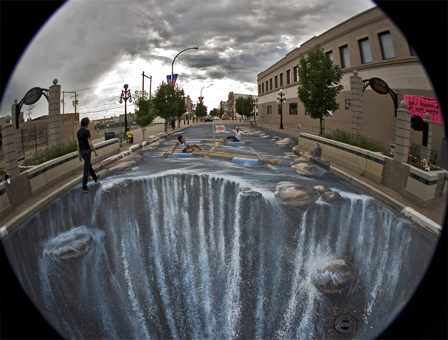This detailed image captures a remarkable piece of 3D street chalk artwork, meticulously crafted to depict a waterfall and river scene on a large parking lot or alleyway in front of a building. The artist has ingeniously manipulated perception, making the water in the foreground appear strikingly real, as though viewers are gazing into a deep pit. The waterfall is painted in vivid blue hues, enhancing the illusion of cascading water.

A person, dressed in black pants and a black short-sleeve shirt, is walking on the left side of the image, seemingly traversing the illusory edge of the waterfall. The scene is set against the backdrop of a rectangular, two-story building on the right, constructed from gray and tan stone. Several streetlights hover over the area, although they are currently turned off.

The photograph itself is taken with a fisheye lens, giving it a circular enclosure against a predominantly black background. This perspective enhances the illusion of depth in the street art, making the entire scene appear even more immersive. The sky in the background is dark and cloudy, adding a dramatic ambiance to the already captivating artwork.